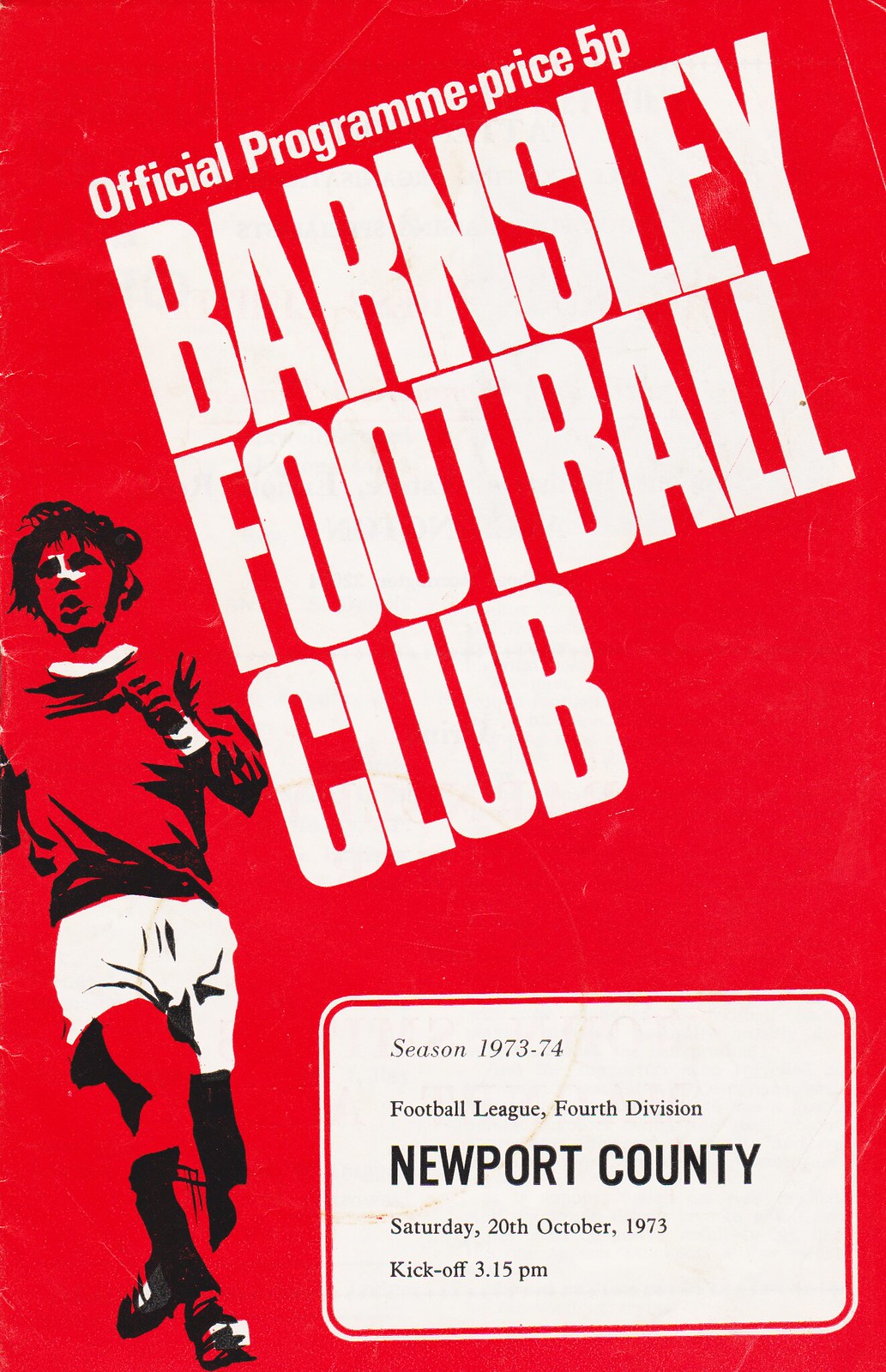The image is the front cover of an official football program for Barnsley Football Club from the 1973-74 season. The background is red, with large white text prominently displaying "Barnsley Football Club." Above this, in smaller white print, it reads "Official Program Price 5P." To the left, there is a detailed drawing of a football player in action, wearing a red jersey and white shorts, with black shading accentuating his features and movement. The player's skin appears red, matching the background, and he has wavy hair and a white streak near his nose. Below the main title, in a white rectangle with rounded corners, it states "Football League Fourth Division Newport County, Saturday 20th October 1973, Kick-off 3.15 p.m." The color scheme of the image is consistent, featuring red, white, and black.